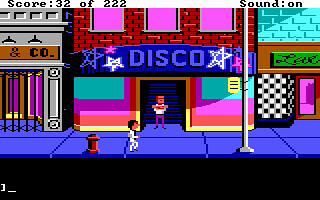A detailed caption for the given image is as follows:

"This pixelated screenshot captures a nostalgic scene from an early-era video game, reminiscent of classic arcade-style graphics. Dominating the image is the front of a building, featuring prominently a sidewalk where a dark-haired character clad in white is walking. The standout feature of this building is a disco establishment, clearly marked by a blue sign overhead that reads 'Disco,' flanked by pink, blue, and white stars on either side. Stationed in the doorway is a gentleman who appears to be a bouncer, lending an authentic touch to the club entrance. Flanking the disco are two other indistinct shops, adding to the urban ambiance. Notable elements include a red fire hydrant behind the walking character and a metal street pole that likely supports a lamp, situated ahead of him. The upper left corner of the image displays the game score as '32/222' in black letters, indicating the player's current achievement. Additionally, the upper right corner confirms that the game is being played with the sound on. The simplistic graphics and limited detail underscore the retro charm and amateurish feel typical of early video game designs."